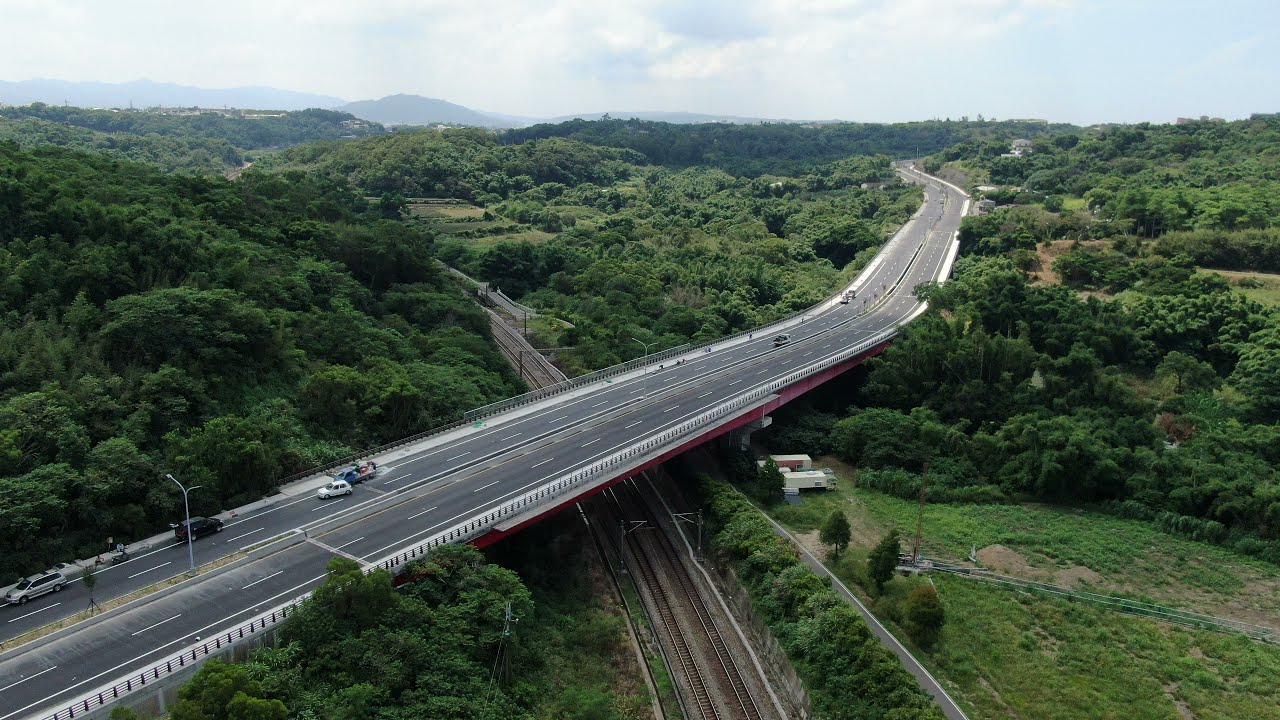This aerial image, likely captured by a drone or helicopter, showcases a four-lane overpass intersecting a set of diagonal railroad tracks, forming an 'X' in the view. The overpass features two lanes in each direction, divided by a thin median with street lamps. Pedestrian paths flank either side of the roadway, which is bordered by fences to prevent vehicles from veering off into the lush, densely packed deciduous trees that fill the scene. A few cars are visible on one side of the road. In the backdrop, a bluish-gray mountain rises subtly above the verdant landscape. The sky above is mostly cloudy with a hazy, gray-blue tint. The entire area gives away an expansive view of greenery extending as far as the eye can see, accentuating the natural beauty surrounding the infrastructure.